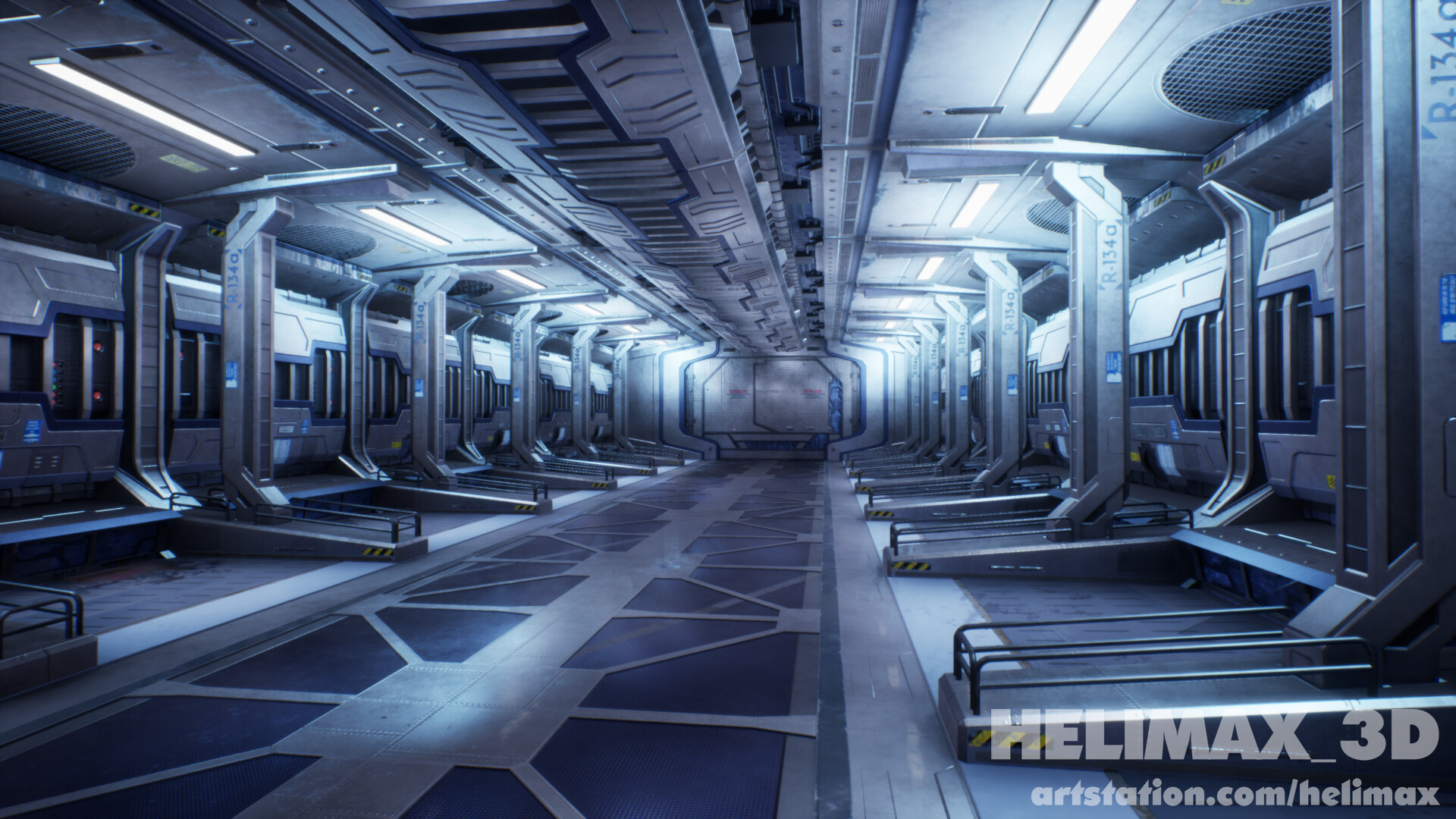The image depicts a detailed 3D-rendered, futuristic metallic corridor or room, potentially the interior of a spaceship or high-tech facility. The environment is characterized by its angular paneling on the ceiling, walls, and floor, all of which give off a sleek, silver-gray metallic sheen. The corridor is lined with evenly spaced columns on both sides, each with small platforms extending toward the center, surrounded by black railings with striped warning markings. The center walkway features a lattice design leading to a large, sliding sci-fi door at the far end. The ceiling hosts several light fixtures, six on each side, interspersed with air vents positioned near the top corners. The bottom right corner of the image features semi-transparent white text reading "Helimax_3D, artstation.com/Helimax," advertising the digital artist's work.